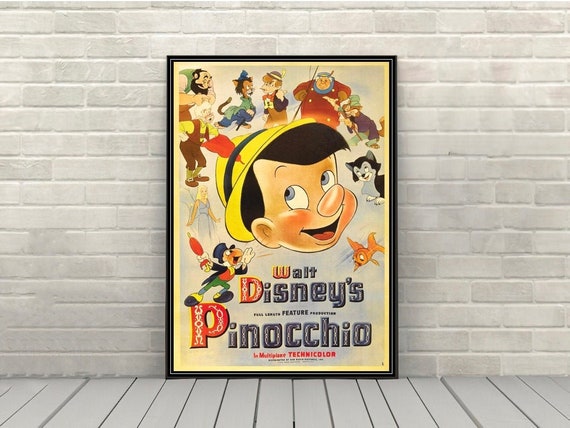This image is a detailed movie poster for "Walt Disney's Pinocchio," propped against a white brick wall and white wooden planked floor. At the center of the poster is Pinocchio, the wooden boy brought to life by a fairy's wish, depicted with brown hair, blue eyes, and a yellow hat adorned with a blue band and a red feather. He's smiling and glancing to his top right. Surrounding him, there's an array of supporting characters: Jiminy Cricket, clutching a red umbrella, leans on the lettering and yells into Pinocchio's ear; an old man with white hair, likely Geppetto; a bald man with a black beard; a goldfish situated to Pinocchio's bottom right; a lady and a cat nearby; and various other characters from the story, including those who try to lead Pinocchio astray, scattered across the top right of the poster. The background has a blue hue, and the poster's border is a striking red. The bottom of the poster prominently features the words "Walt Disney's Pinocchio" in red and black letters, along with "Technicolor" beneath it.